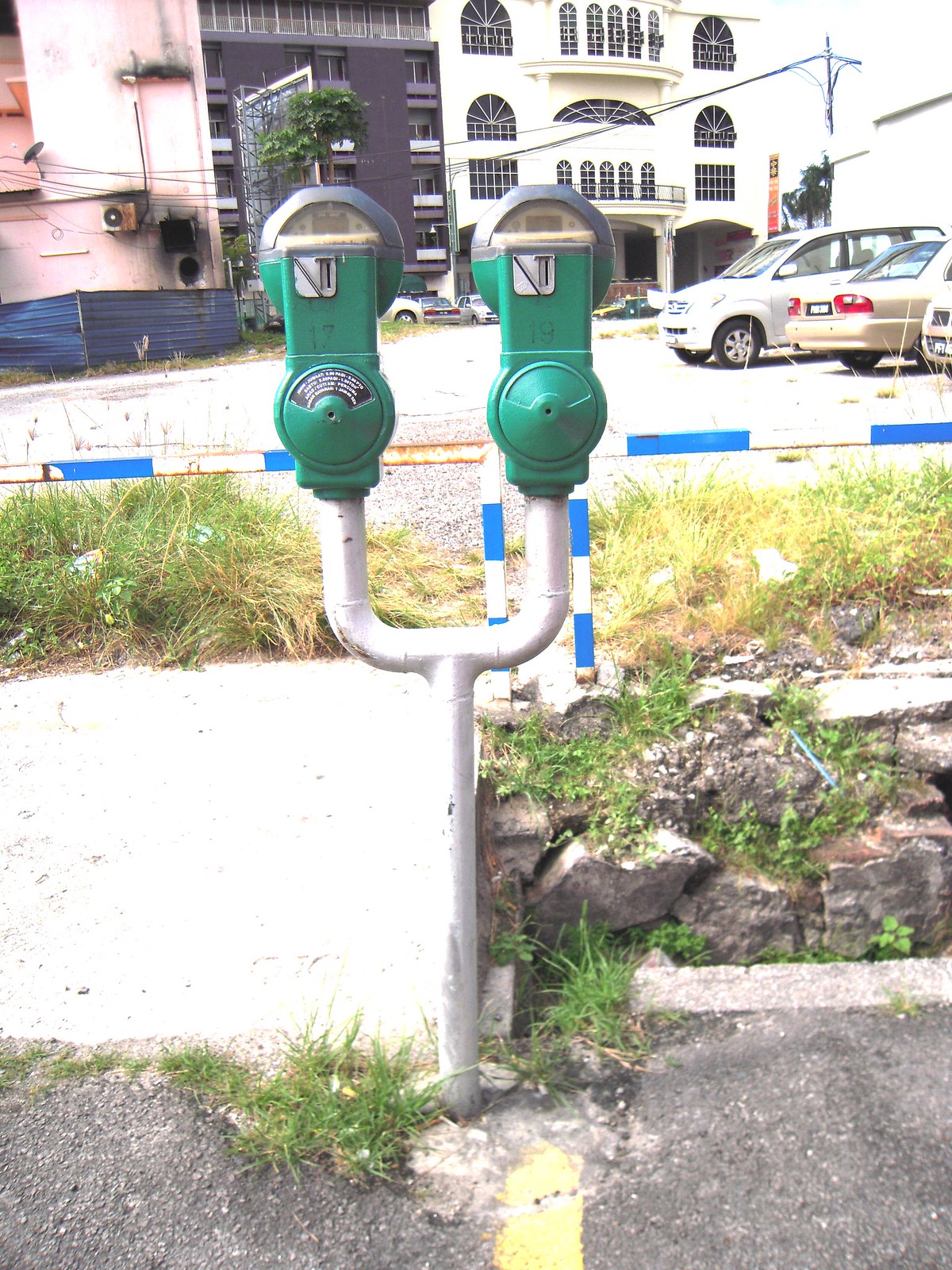The image showcases a vintage parking meter positioned centrally but slightly to the left within a taller-than-wide frame. Approximately 15% up from the bottom, a white pole emerges from a pavement lined with a yellow stripe, extending vertically for about 40% of the image before splitting into two perpendicular pipes. These pipes support dual green parking meters with gray tops, marked as "17" and "19," featuring silver coin slots. Directly behind the meters, the parking lot with two marked spots is visible, interspersed with patches of grass and rocks. In the background, a sequence of tall buildings rises, including an adjacent white building with black windows, a black building, and a pink building. Several vehicles are parked nearby, notably a silver van and the rear segment of a brown car, along with a distinct blue and silver horizontal pole.